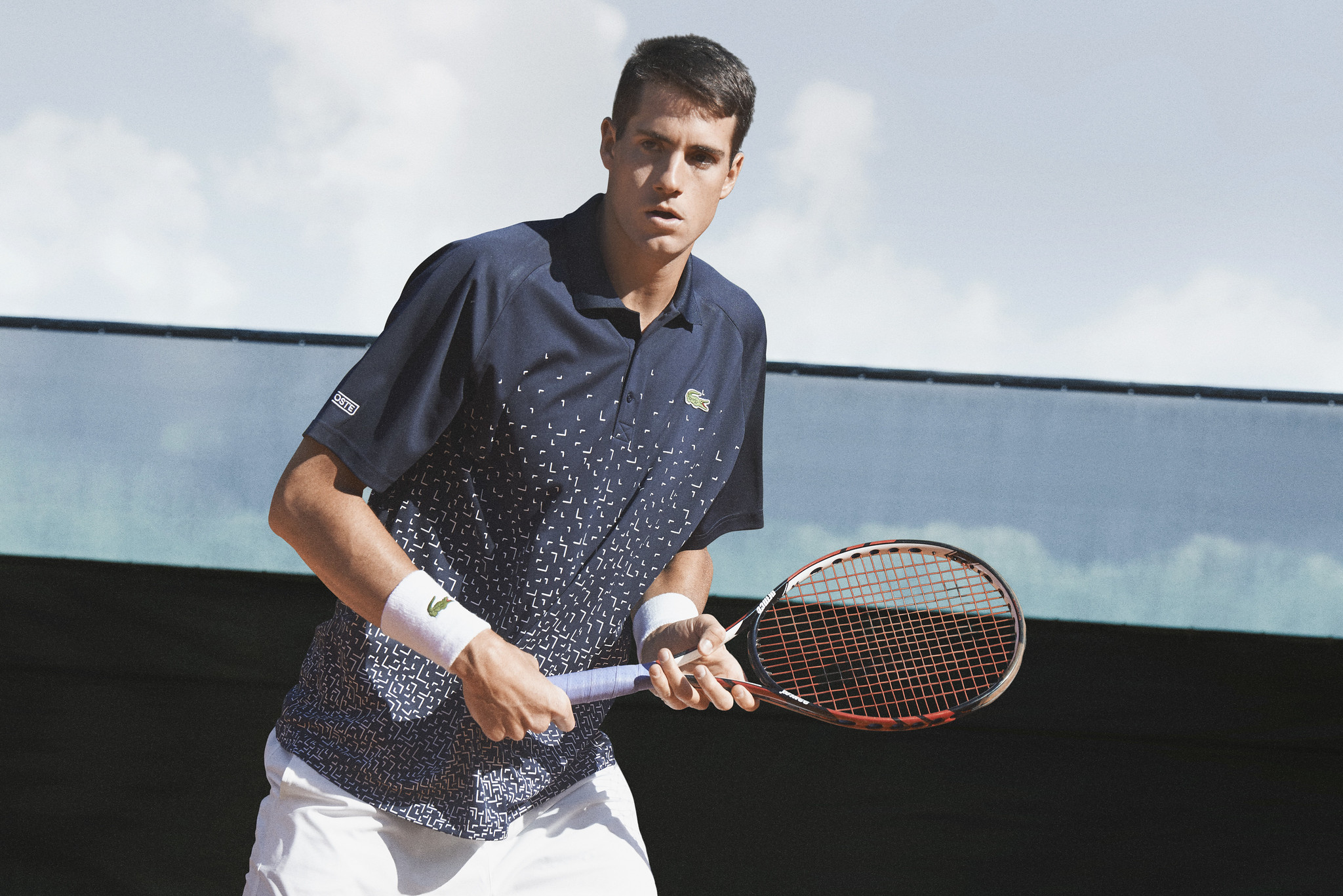The photograph captures a male tennis player, seen from his upper calves to the top of his head, as he intently focuses on the game. He sports a blue, short-sleeve polo shirt adorned with white patterns resembling falling leaves or speckles. The shirt features an unbuttoned collar with two buttons, and a green Lacoste crocodile logo on the top right. His white pants complement white wristbands on both wrists, which also display the Lacoste crocodile logo, adding to his coordinated athletic appearance.

In both hands, he grips a distinctive tennis racket with a black, orange, and white rim, an orange net, and a gray-wrapped handle, suggestive of his readiness to strike. The player has short brown hair that’s longer on top and shorter on the sides and wears a focused, serious expression. His tanned skin catches sunlight on the right side of his face, while casting shadows on the left.

Set against a background comprising a blue and black see-through tarp with subtle white clouds visible both through and above it, the upper third of the scene reveals a partly cloudy sky, light gray with multiple white clouds. The photograph, horizontally aligned and rectangular, exudes a vintage feel, reminiscent of the late 70s or early 80s, showcasing both the player's intensity and the timeless appeal of the sport.